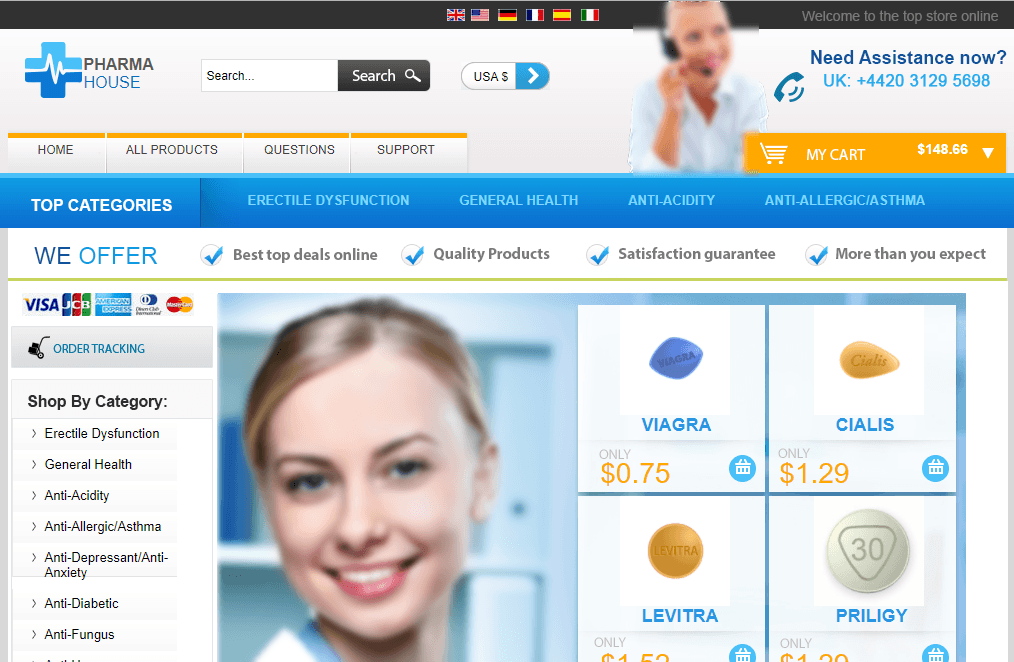The image is a screenshot from the website "Pharma House." The logo, positioned at the top-left, features "PHARMA" in navy and "HOUSE" in teal, with a distinctive plus sign in the same colors, containing a white heartbeat symbol at its center.

To the right of the logo is a search bar, marked with a magnifying glass icon, inviting users to browse the site. Next to this is an image of a customer service representative, either a man or woman, wearing a headset and appearing ready to assist. Below this image, text reads, "Need assistance now?" followed by "UK" and a contact phone number.

Adjacent to the customer service section is a cart icon displaying a monetary total of $148.86. Above this area, navigation links are prominently displayed: "Home," "All Products," "Questions," and "Support."

Below the navigation menu, there is a "Top Categories" section listing various product categories: "Erectile Dysfunction," "General Health," "Anti-Acidity," "Anti-Allergic," and "Asthma." The website also highlights its key offerings with blue check marks: "Best top deals online," "Quality products," "Satisfaction guaranteed," and promises "More than you expect."

Further down, there is an image of a female pharmacist surrounded by four different types of pills, suggesting the variety of products available for selection.